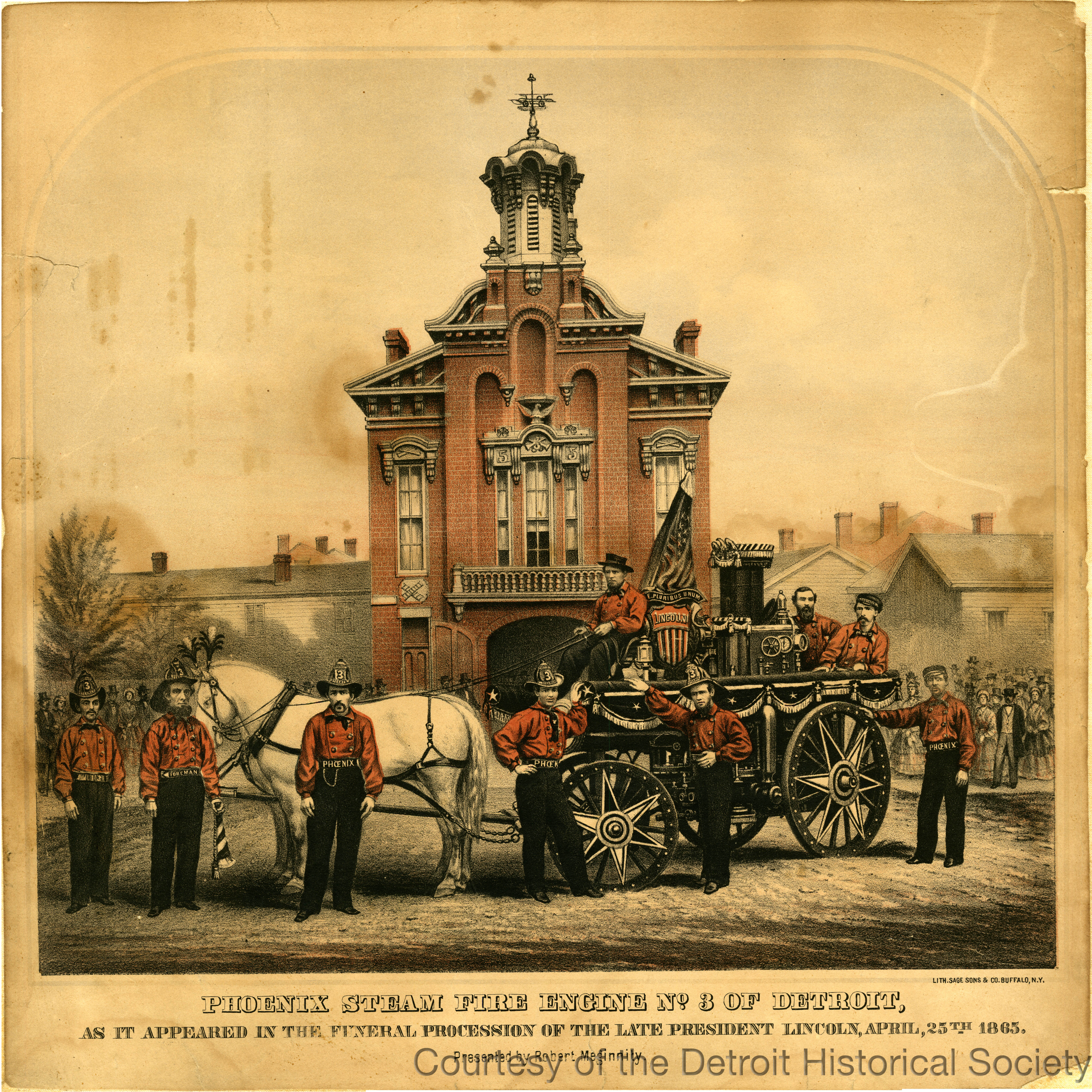This detailed painting, courtesy of the Detroit Historical Society, depicts the Phoenix Steam Fire Engine No. 3 of Detroit as it appeared in the funeral procession of President Lincoln on April 25, 1865. Set against an overcast sky, the image centers on a stately red brick building with a gray balcony and trusses. The scene is bustling with approximately ten firefighters in distinctive red vests, black pants, and traditional fire helmets, some featuring the number 3. The central focus is a white horse-drawn steam fire engine with large wheels adorned with star-shaped spokes. The firefighter at the reins is dressed in a red vest, black pants, and a small top hat, holding a tattered American flag. In the background, a mix of gray-roofed buildings and a church spire rise, with chimneys and trees scattered throughout. Additional figures include bearded men and those with handlebar mustaches, some slightly obscured by smoke, all contributing to the historical ambiance. The aged beige wall behind adds to the illustration's antiquity, reinforcing its historical significance.